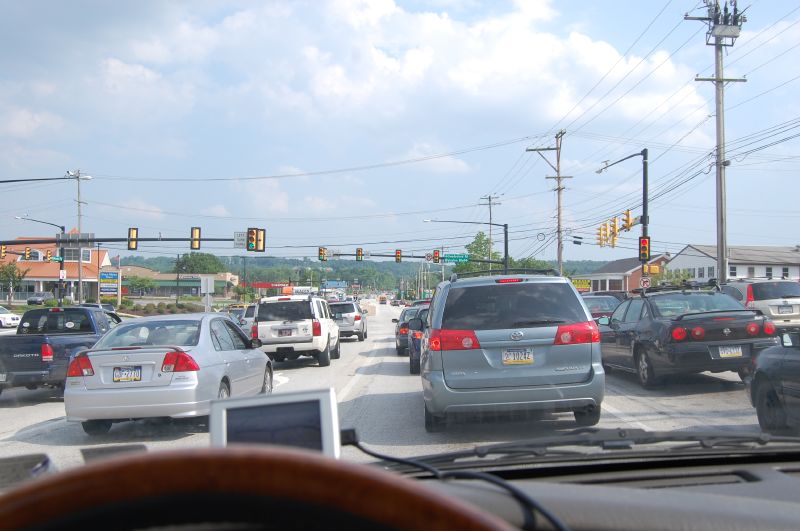A photograph taken from inside a car showcases a bustling urban street scene. The bottom portion of the image reveals the car's brown steering wheel, hinting at the perspective of a driver. Outside the windshield, the view expands to a busy street where multiple cars are halted at a traffic light. The street is divided into four lanes, all filled with vehicles heading in the same direction. Black-posted traffic lights hang overhead, contributing to the urban infrastructure. The sky above is a serene blue, punctuated by scattered white clouds. Distant trees, displaying a mix of green and brown foliage, add a touch of nature to the scene. Flanking both sides of the road are various buildings, further illustrating the city's bustling environment.